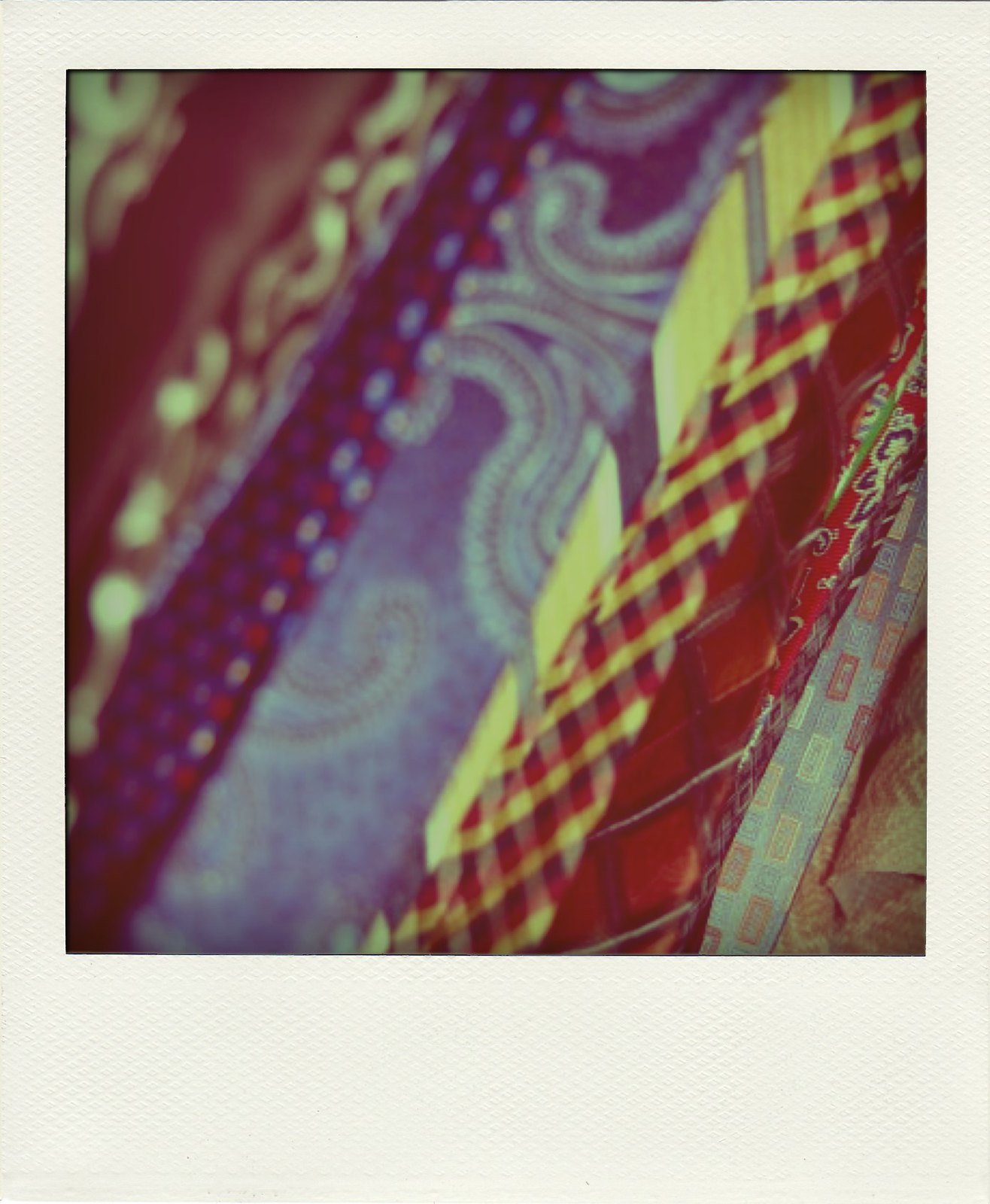The vintage Polaroid picture, framed with white edges and featuring a rectangular shape with a thicker bottom border, captures a slightly blurred close-up of a series of neckties arranged side by side. The ties, presented in a diagonal pattern across the image, display a variety of colors and patterns, ranging from blue, navy, light blue, yellow, red, black, gray, brown, to purple. The left-hand side of the picture is extremely blurry while the right-hand side appears clearer. Each tie boasts a unique design, including paisley, checkerboard, plaid, vertical rectangles, polka dots, X’s, diamonds, and abstract shapes. A yellowish tinge permeates the photo, lending it a dated and nostalgic feel reminiscent of early Instagram shots from 2012. The combination of faded colors and various patterns on the fabrics highlights a mix of gingham stripes, burgundy with circles, and gray ties with red, white, and orange squares, creating a visually rich and textured composition.